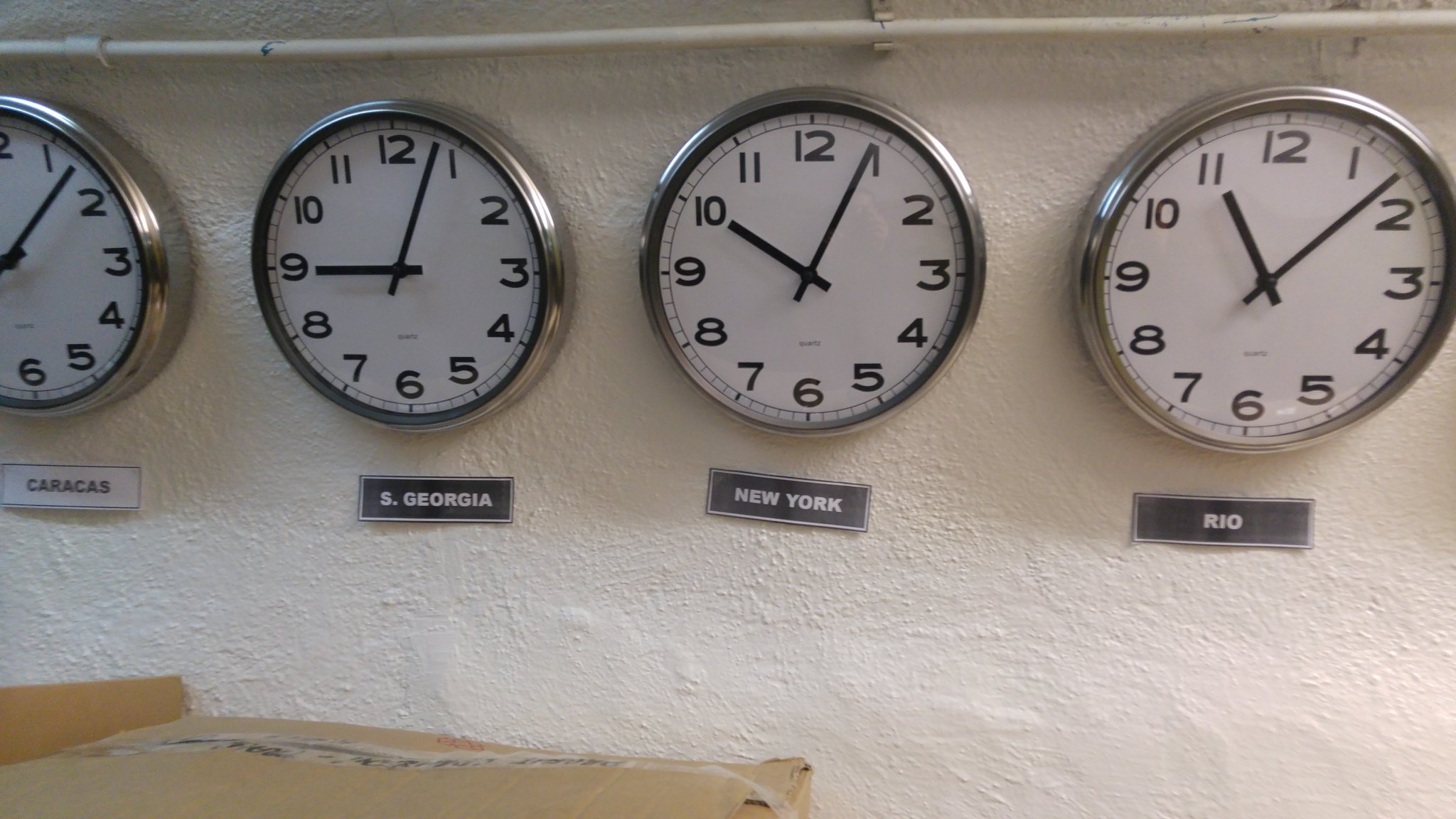This image captures a series of four analog clocks mounted on a gritty, white stone wall. Each clock has a white face with big, bold black numbers, black hour and minute hands, and silver edges. The clocks are arranged in a row from left to right, and each one is labeled underneath with the respective city it represents. The first clock, partially visible, represents Caracas and appears to show a time around eight minutes past. The second clock, labeled "S. Georgia" with a black plaque, displays 9:03. The third clock, marked "New York" also with a black plaque, shows 10:04. The fourth clock, under the label "Rio" with another black plaque, indicates the time as 11:07. Above the clocks runs a long pipe or handlebar, and below the first clock on the left-hand side, there is a brown box.